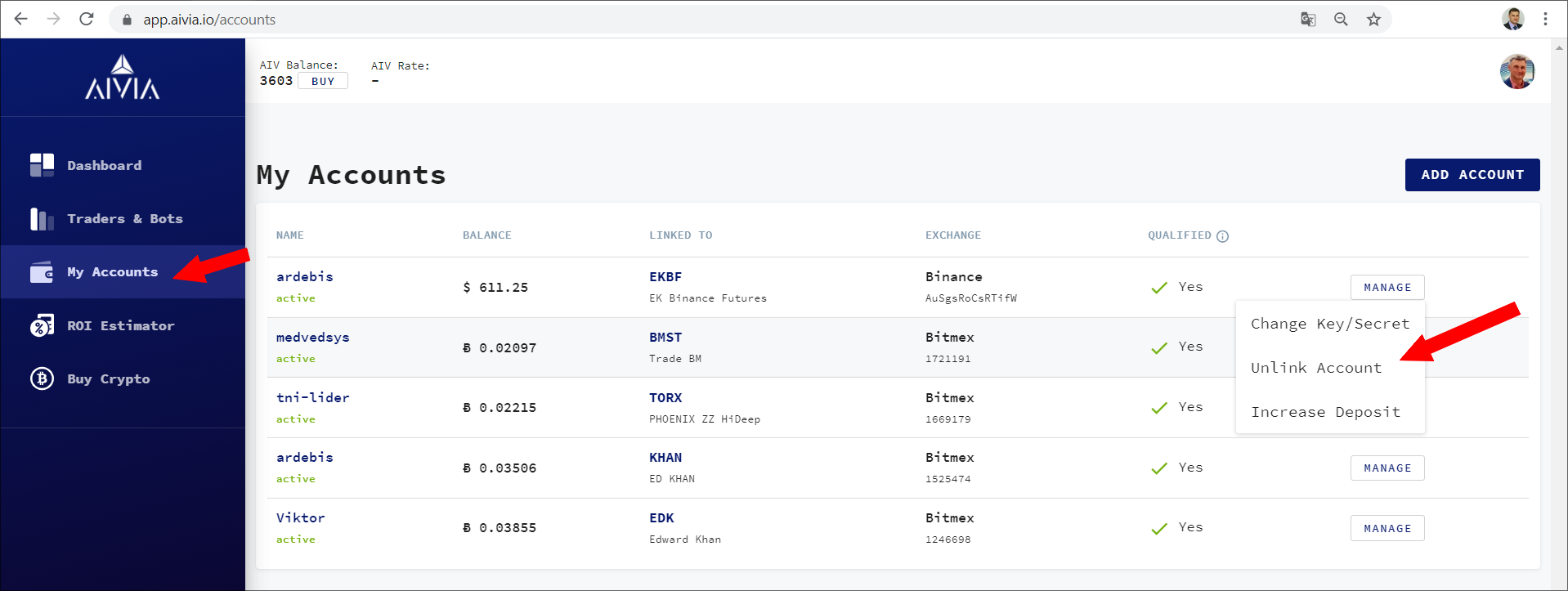In the screenshot of the AIVIA platform's webpage, the URL displayed in the address bar at the top reads "app.aivia.io/accounts." The left-hand side features a dark blue sidebar with the company logo at the top. The logo, designed in white, consists of three half-triangles forming a larger triangle. Below the logo, the brand name "AIVIA" is written in white capital letters. The sidebar menu lists several options: "Dashboard," "Traders and Bots," and "My Accounts," the latter being highlighted with a solid red arrow pointing towards it. Other menu options include "ROI Estimator" and "Buy Crypto."

The main content area has a white background. At the top, next to the company logo, in a dark, thin font, are the labels "AIV Balance:" and "AIV Rate." Beneath the "AIV Balance" label, the number "3603" is prominently displayed in bold black font. Adjacent to this, there is an all-caps button labeled "BUY."

Further down, in a large, bold black font, the heading "My Accounts" is displayed. Below this heading, five columns are arranged in a blue-highlighted row with the titles "Name," "Balance," "Linked To," "Exchange," and "Qualified." Within the "Linked To" column, the mouse cursor is visible. The accounts list below the header includes various details such as account names, balance amounts, linked companies, exchange rates, and qualification statuses. Each qualified status is indicated with a green checkmark followed by the word "Yes."

To the right of the account details, there is another section featuring options like "Change Key/Secret," "Unlink Account," and "Increase Deposit," with a solid red arrow pointing to the word "Account" within "Unlink Account."

Above this section is a dark blue banner button labeled "ADD ACCOUNT" in white uppercase letters. At the very top-right corner of the webpage, there is a profile picture of the account owner, an older gentleman of European-Caucasian descent.